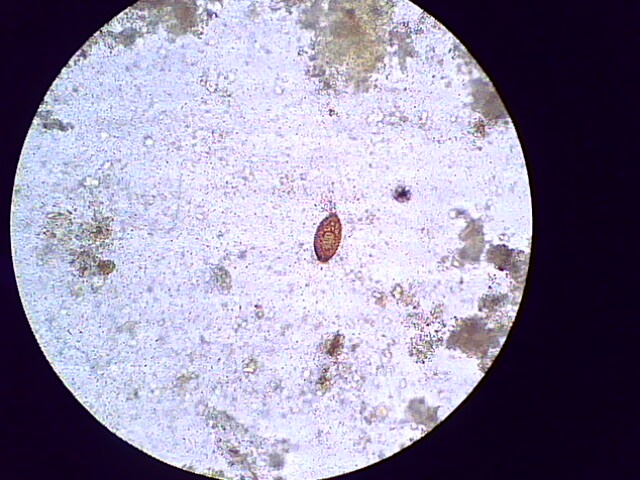The image appears to be a close-up view through a microscope, featuring a large white circular field encased within a black rectangular background. Predominantly occupying this circular field is a chalky white surface scattered with specks of various colors. Toward the center-right, there is an elliptical or oval-shaped object with red and brown patterns, potentially resembling a crab shell or a single-celled organism such as a cell or a microorganism. This central object has indistinct edges, making it difficult to ascertain its exact nature. Surrounding the main object, there are several irregularly shaped blobs in colors ranging from blue-gray to green and brown, particularly concentrated at the top and right edges of the circle. The scene is dominated by the intricate textures and subtle color variations of the white surface and its surrounding elements, invoking a sense of magnified biological or geologic material.